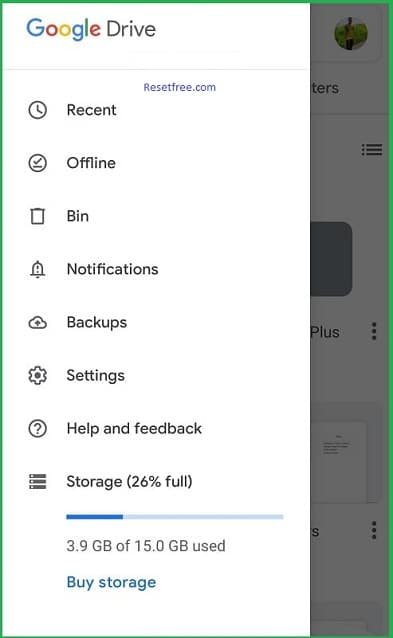This cropped screenshot provides a detailed view of the Google Drive interface, focusing on the options tree panel to the left. At the top left of this panel, the Google Drive logo is prominently displayed, featuring the Google logo followed by the word "Drive" in gray. Below this, various categories are listed in a vertical sequence: Recent, Offline, Bin, Notifications, Backups, Settings, Help & Feedback, and Storage.

The storage section shows that 26% of the allocated space is used, represented by a progress bar indicating 3.9 GB of 15 GB being used. At the bottom of the panel, there is a centered "Buy Storage" button in light blue.

In the background, the main Google Drive interface is visible but grayed out due to the open tab tree. The user's profile picture is located in the upper right corner of the background area, providing a sense of personalized account details. This detailed breakdown captures the various functionalities and the interface layout of Google Drive.